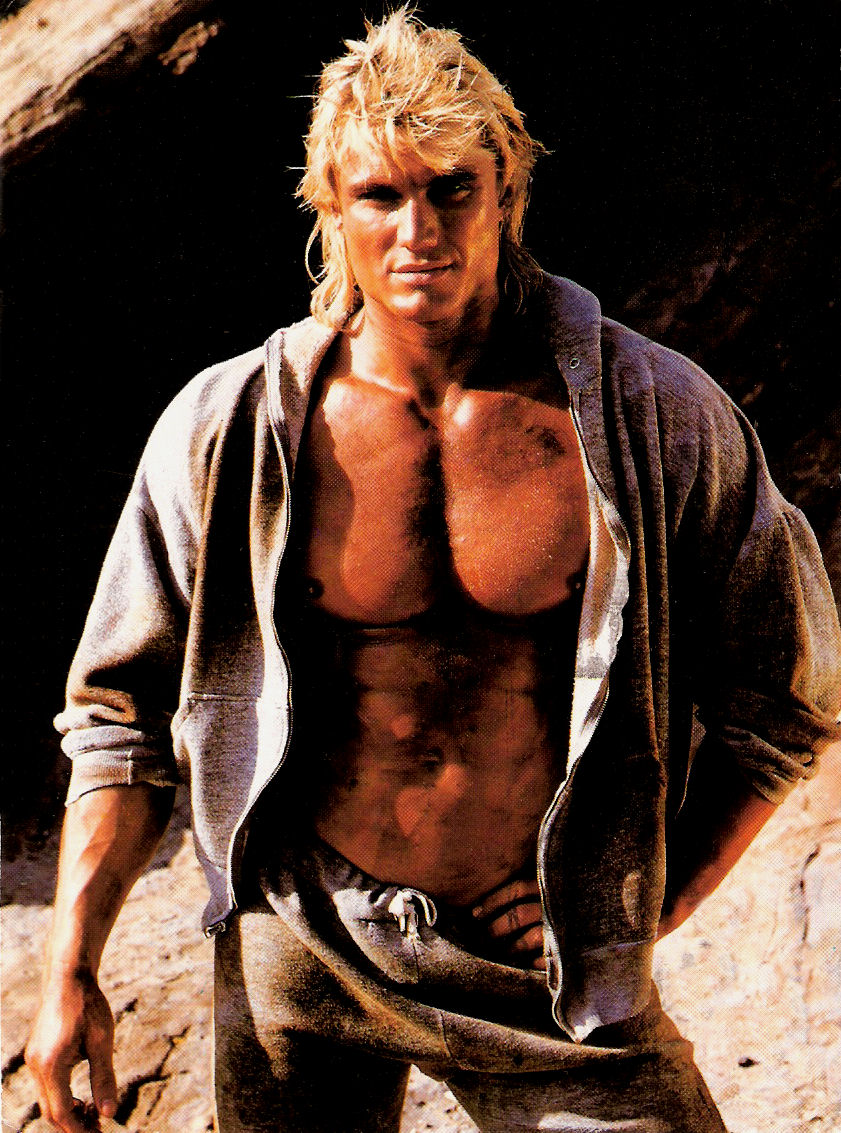A man with disheveled blonde hair cascading down to his right shoulder and likely extending behind his head stands facing the camera directly. He wears a gray jacket with sleeves rolled up, exposing his shirtless torso and well-defined abs. His right arm hangs casually by his side while his left arm rests at his waist. Below, he sports gray sweatpants that appear rather dirty. His expression is neutral, eyes fixed on the camera. The background features a small, slate-colored rock in the upper left corner, with a predominantly black backdrop and a rocky, dirt-covered ground, suggesting he might be in a cave, possibly for a movie shoot.